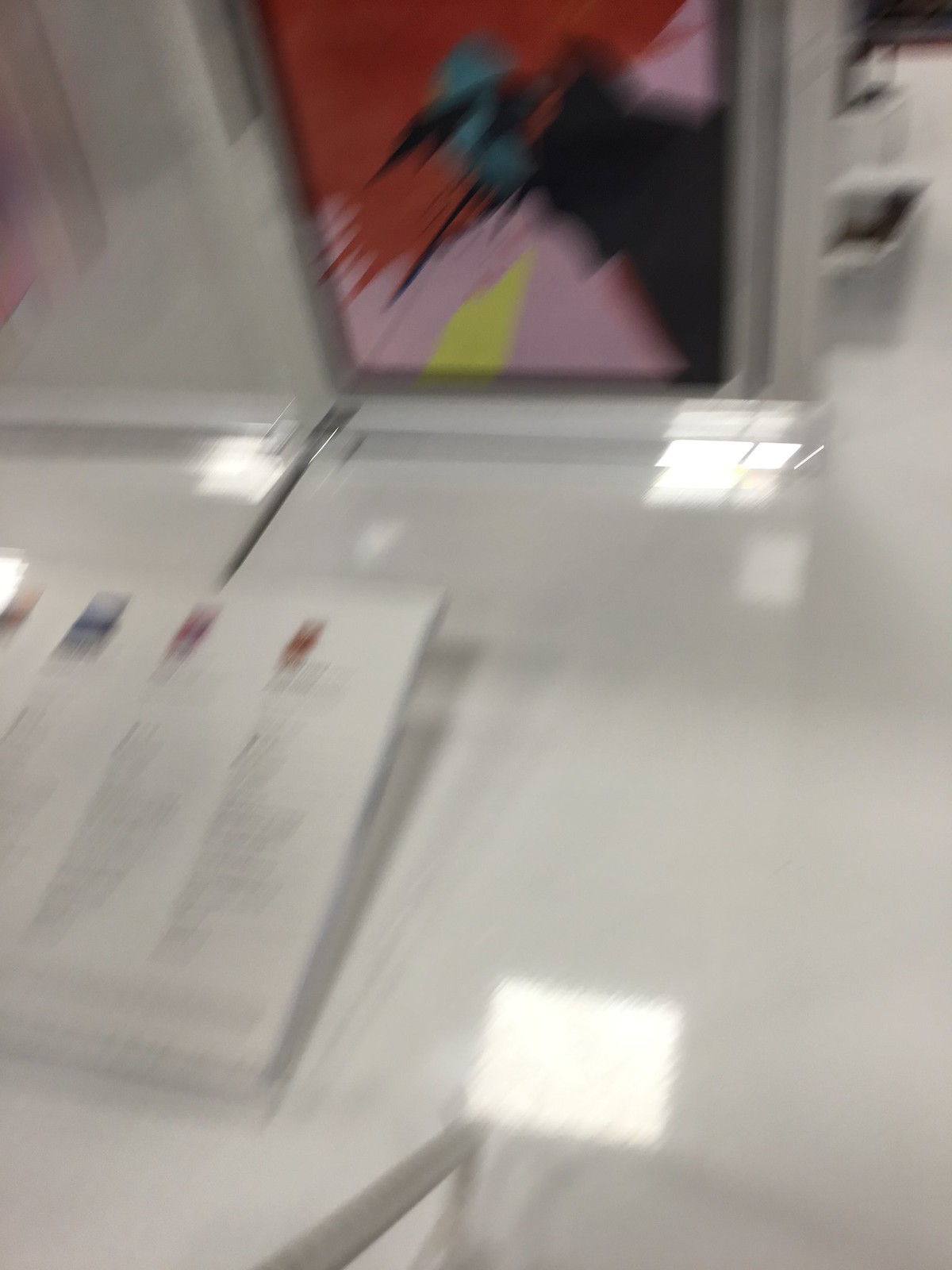The image depicts a blurry scene likely taken in a store, museum, or educational facility. Central to the composition is an abstract painting or art piece. Dominating the artwork is a diagonal swath of red stretching from the top left to the bottom right, bordered by pink hues and intersected by a streak of yellow. Complementary blue and black elements form jagged lines mid-painting, resembling a bird’s head. The painting, standing upright with a grayish-black bezel or frame, is displayed on a shiny white surface, possibly a table. A paintbrush with blue or black on its bristles points towards the painting, emerging from a white packet filled with brushes. Nearby, a long piece of angled paper or a sign describes the object on display. In the background, a thin, transparent glass holder, a cabinet or shelf, and potentially the arm of a chair or a short staircase are visible, adding to the scene's dynamic and cluttered nature.